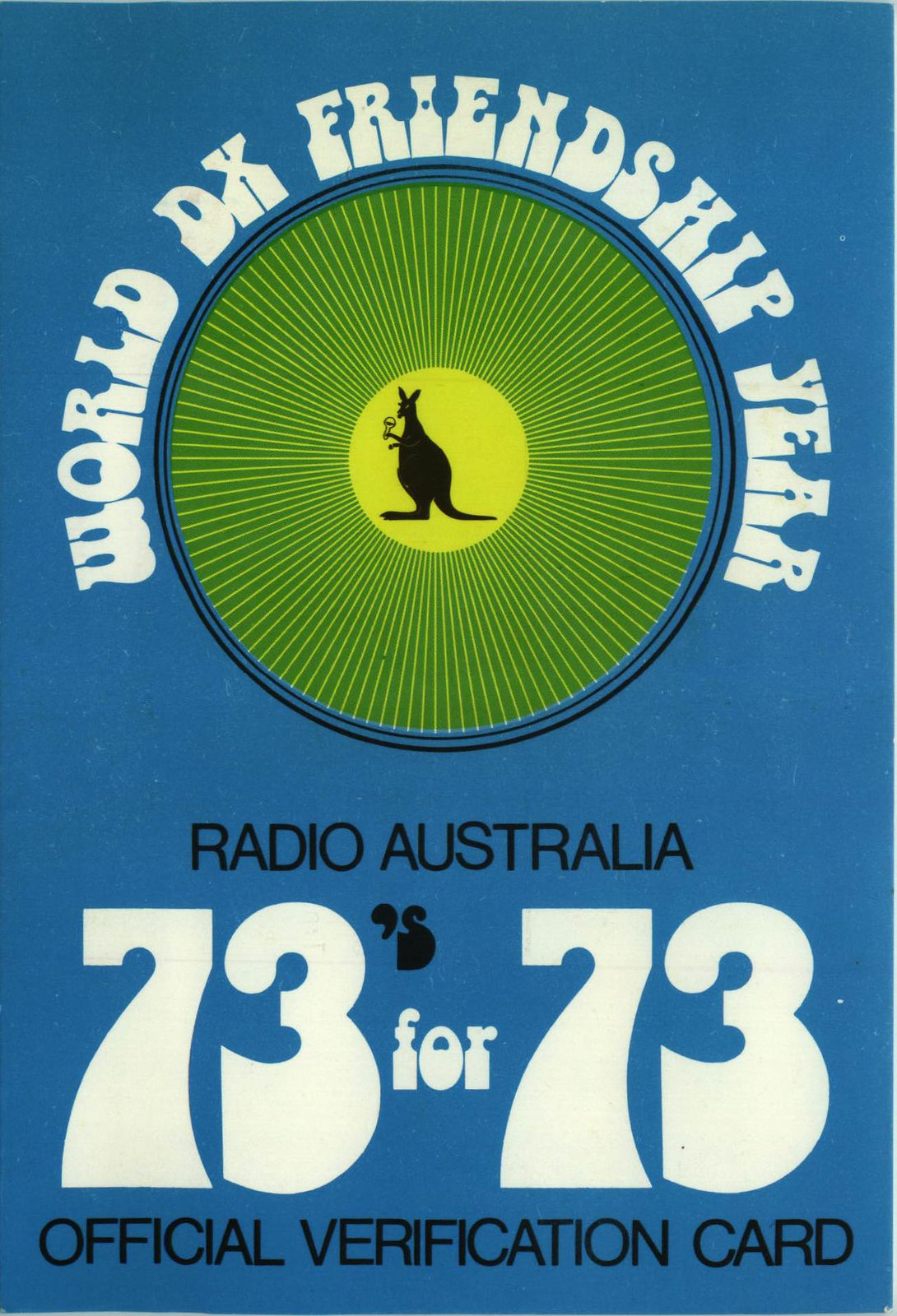The image features a vertically-oriented rectangular poster or card with a blue background, prominently showcasing an official verification card for an event. At its center is a large blue circle, within which is a smaller yellow circle depicting a kangaroo. Radiating outward from the yellow circle are green and yellow lines that extend to the blue frame. At the top, curved around the circle, it reads "World DX Friendship Year." Beneath that, in bold black capital letters, is "Radio Australia," followed by the text "73s for 73" in white letters. The bottom of the card bears the words "official verification card." The primary color scheme includes blue, black, white, green, and neon green.